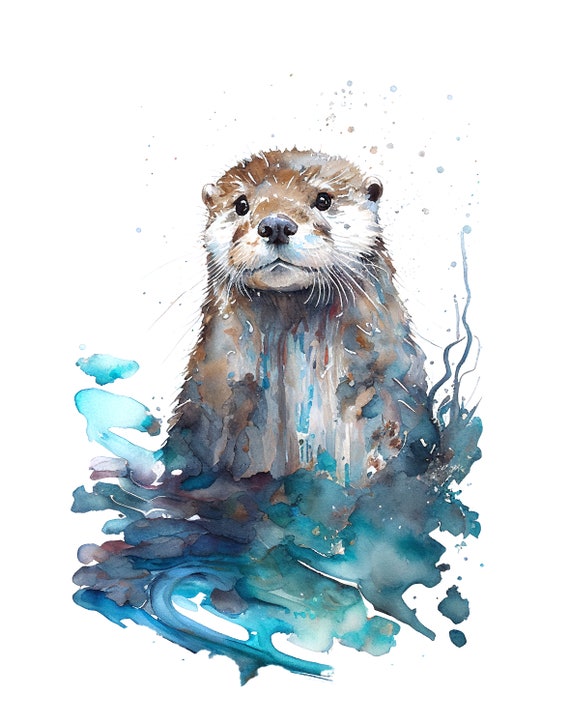The image is a detailed painting of an adorable otter, partially submerged with about half of its chest out of the water, looking directly at the viewer. The otter's head is brown, adorned with small, round ears, dark eyes, a black nose, and prominent white whiskers. The fur under its eyes and around the cheeks is white, providing a striking contrast to its otherwise brown face. Below the neck, the painting transitions into a more abstract style, where vibrant splashes of blue, white, and red blend seamlessly on its chest, giving the appearance of watercolor smears. The water around the otter features an array of colors, including aqua blue, purple, dark blue, and green, further enhancing the dreamy, artistic quality of the artwork. The background is clean white, accented with a few beige and blue dots, making the central figure stand out even more. This charming piece showcases intricate detail, particularly in the otter's expressive face, and could be a perfect design for prints, stationery, or wildlife-themed art collections.